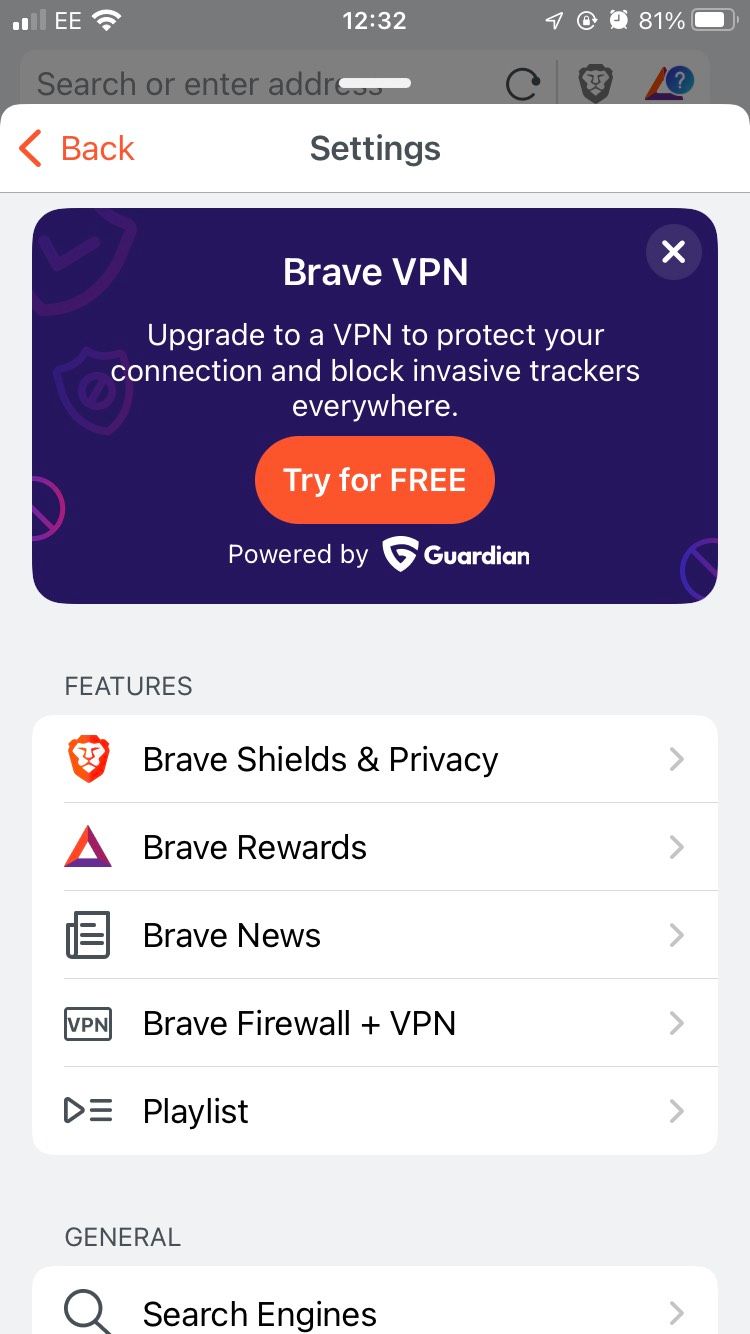This screenshot from an iPhone captures various elements on the screen, starting with the status indicators at the top. In the top left corner, there are two out of four data bars, with the first two bars filled in white and the remaining two in gray, suggesting an ascending pattern in signal strength. Adjacent to the data bars are two capital 'E's indicating extended service. Following this, a white Wi-Fi symbol is visible.

Centrally located in the status bar, the time is displayed as 12:32. Proceeding rightward, a navigation icon points towards the right, followed by a rotate lock symbol. An alarm clock icon is next, alongside an 81% battery indicator, where the battery icon is mostly filled.

The main part of the image shows an open settings menu. On the left-hand side, there's an orange back button with an arrow pointing to the left. Centered at the top in black text is the word "Settings."

Beneath this, there is what appears to be an advertisement, roughly the size of a credit card, featuring a promotional banner for Brave VPN. This section has a dark purple background adorned with various pink and purple images, including shields, circles with lines through them, and a shield bearing a checkmark. At the top center, 'Brave VPN' is inscribed in white text. Below, in smaller white text, it reads: “Upgrade to VPN to protect your connection and block invasive trackers everywhere.”

At the bottom of this promotional section is an orange oval button with the text "TRY FOR FREE" in capitalized white letters. Below this button, it says "Powered by Guardian" with a stylized triangular 'G' representing the Guardian logo, in bold white lettering.

Below the advertisement is a features menu, with each option listed in gray capitalized text and accompanied by a gray arrowhead pointing to the right to signify the presence of further submenus. The listed options are:
1. Brave Shields and Privacy
2. Brave Rewards
3. Brave News
4. Brave Firewall + VPN
5. Playlist